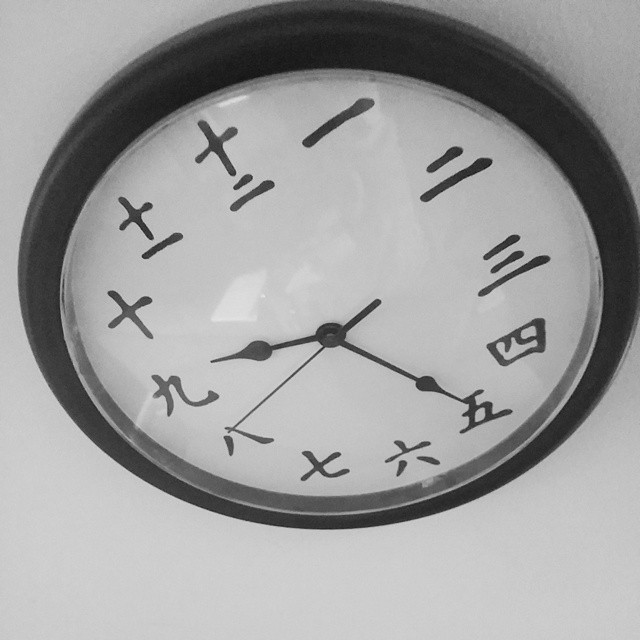A detailed image caption could be:

"A photograph captures a uniquely designed clock mounted on a white wall. The clock features a plain design with a slightly bulging crystal cover and a black outer rim. Its face is adorned with black numbers written in an Asian script, adding an exotic flair. The absence of minute markings between the numbers contributes to its minimalist aesthetic. The clock's minute and second hands are present, though there are no additional markers for precise time reading. The image is taken from a slightly elevated perspective and the clock appears to be slightly tilted counterclockwise. The distinctive numerical style and the clock's overall simplicity make it a standout piece."